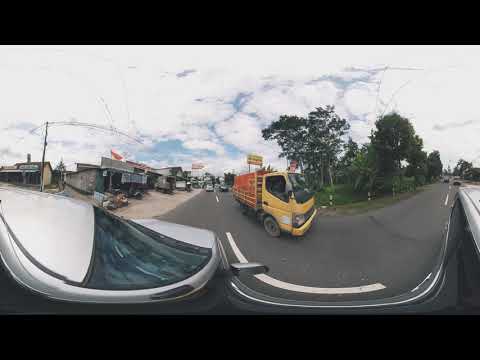This image captures the view from inside a vehicle driving down a two-lane road, taken with a fisheye lens that creates a distorted perspective. On the right, there's a distinctive yellow truck with an orange bed, likely a work or farm truck, heading towards a bend in the road. The road curves around a grassy median dotted with small green trees, suggesting it's taken in spring or summer. The sky is mostly cloudy with patches of blue peeking through, casting a neutral, grayish tone over the scene. To the left, there's a continuation of the road accompanied by a sidewalk and several older one-story buildings or stores. Additional vehicles can be seen both in front of and behind the main vehicle, contributing to the bustling atmosphere of this daytime scene. A light post stands nearby, adding to the urban setting.